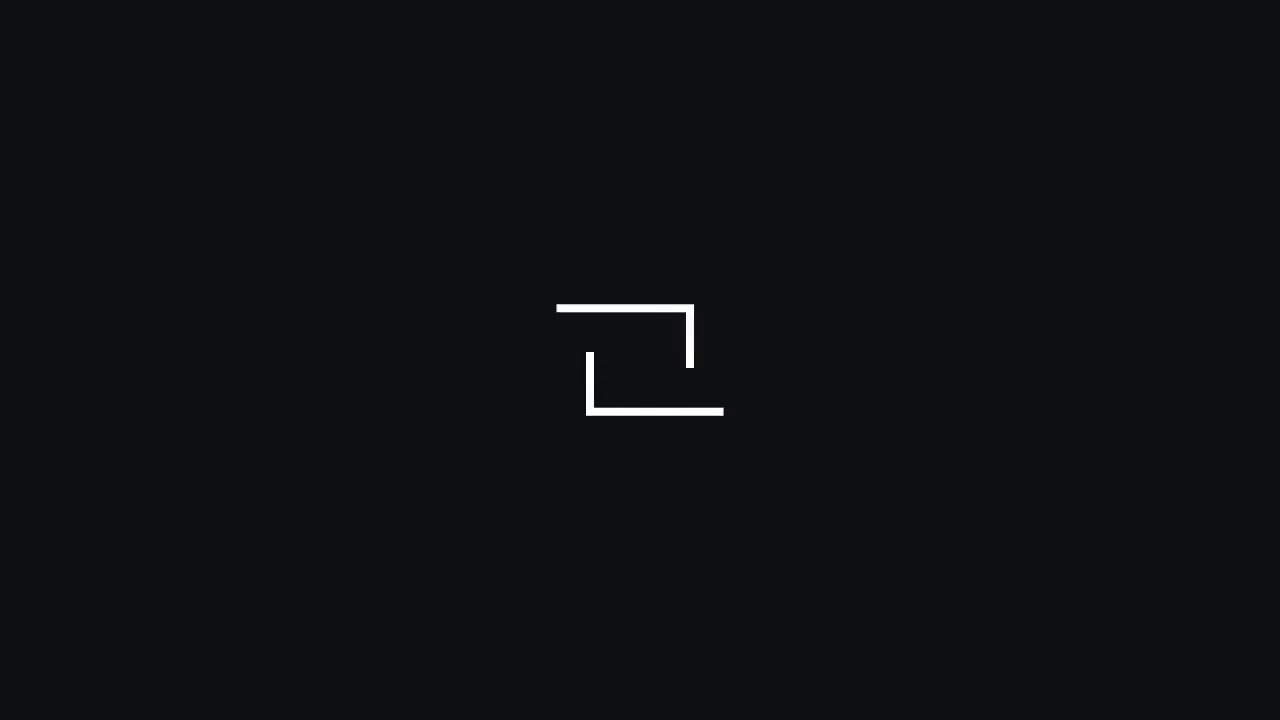The image features a solid black background with no variations in color. In the very center of the image are two thin, white, L-shaped figures. These L-shapes are identical in size and face each other horizontally. The upper L extends horizontally from left to right and then vertically downwards on the right to form the base of the L. Conversely, the lower L extends horizontally from right to left and then vertically upwards on the left to form the base of the L. The L-shaped figures do not touch but are positioned close together, creating a symmetrical and balanced appearance against the stark black background.